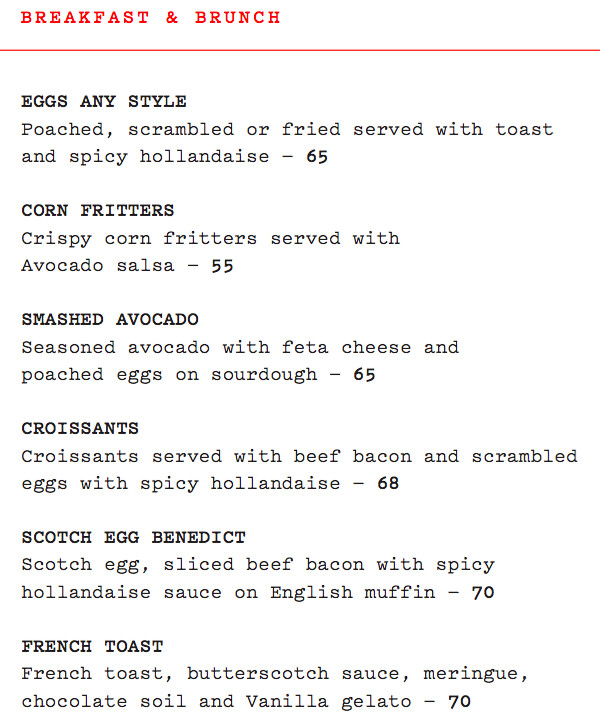In this image, we are presented with a colorful breakfast and brunch menu dominated by shades of red, black, and white. The menu, which occupies the entire screen, starts with various styles of eggs—poached, scrambled, or fried—served with toast and spicy hollandaise sauce. Next, it features crispy corn fritters accompanied by avocado salsa. There's a dish of seasoned smashed avocados paired with feta cheese and poached eggs on sourdough bread.

Continuing, the menu lists croissants served with a combination of beef, bacon, and scrambled eggs draped in spicy hollandaise. Another hearty option is the Scotch egg benedict, consisting of Scotch eggs, sliced beef, bacon, and spicy hollandaise sauce on an English muffin. For those with a sweet tooth, the French toast is a decadent choice, topped with butterscotch sauce, meringue, chocolate soil, and vanilla gelato. The style and layout of this menu make it typical of what you’d expect to find at a cozy breakfast restaurant.